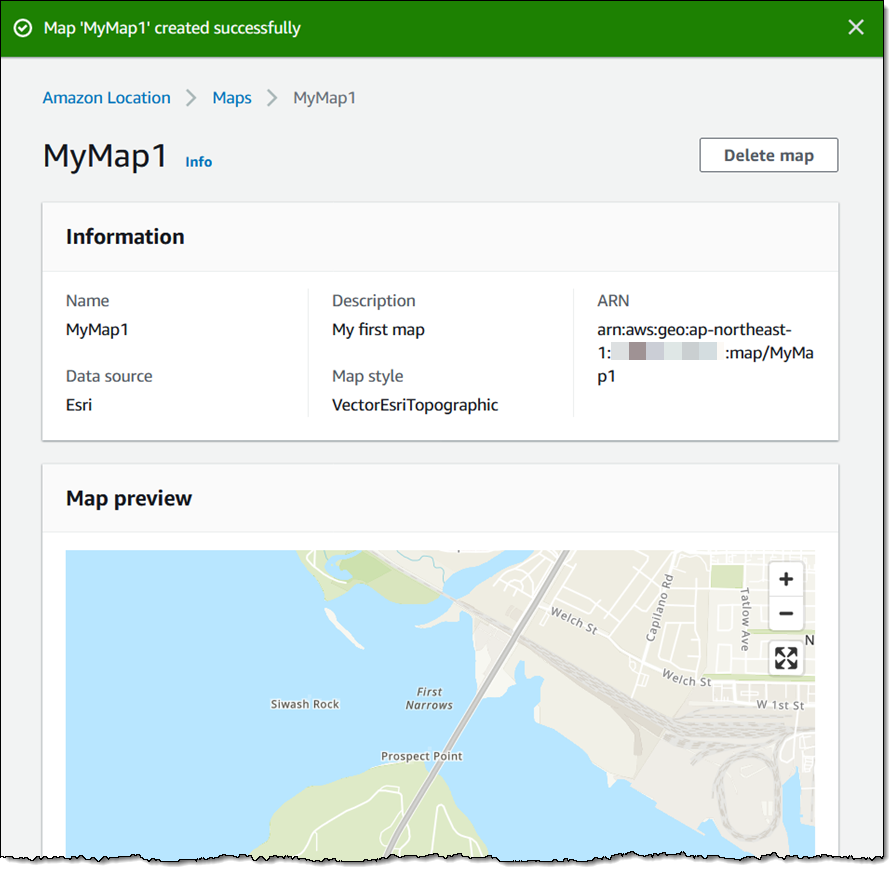This screenshot captures the interface of an app displaying the successful creation of a map named "MyMap1." 

In the upper left corner of the screen, the word "Map" is shown, signifying the section of the app being viewed. On the upper right corner, there is an "X" icon to close the screen. Below the header, the text "Amazon Location" is visible, followed by a breadcrumb trail: "Maps > Map1 > MyMap1."

Immediately beneath this navigation bar, there are options for "MyMap1 Info" indicated by a blue hyperlink, along with a "Delete Map" button situated on the right. 

The "Information" section follows, detailing the map's attributes as:
- **Name**: MyMap1
- **Data Source**: ESRI
- **Description**: MyFirstMap
- **Map Style**: Vector, ESRI, Topographic

On the right side of this information panel, there's a string identifying the Amazon Resource Name (ARN), partially redacted as: "arn:aws:geo:ap-ne:1:redacted:map/MyMap1."

Below this information is a map preview, constituting the lower half of the screenshot. The preview displays an actual map, though the specific geographical area depicted remains unidentified.